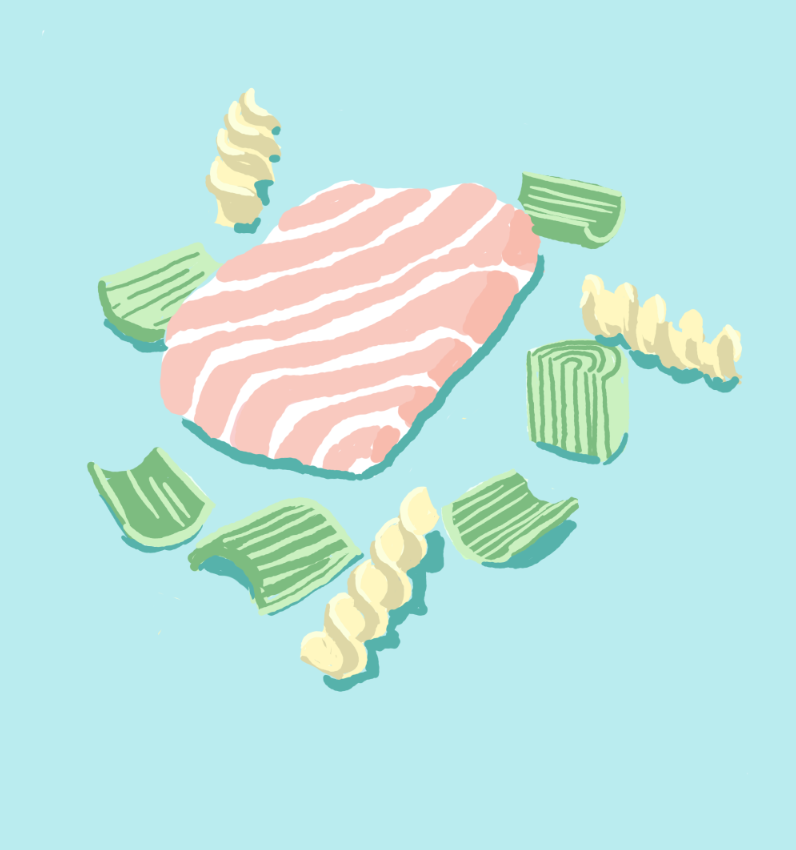This detailed illustration, set against a pale turquoise background, depicts a colorful array of food items in a cartoon style. At the center is a piece of salmon, unmistakably characterized by its pink hue and marbled white lines, giving it a realistic texture. Surrounding the salmon are three pieces of fusilli pasta, illustrated in shades of white and gray, curling like little spirals and thoughtfully positioned in the upper left, right hand side, and bottom right corners. Additionally, six pieces of pale green celery, accented with darker green for texture, are scattered around the fish. These pieces are arranged in various orientations, with some lying flat while others stand upright, adding a dynamic flow to the composition. The overall lighting suggests a light source from the upper left, casting gentle shadows and giving depth to the illustration.